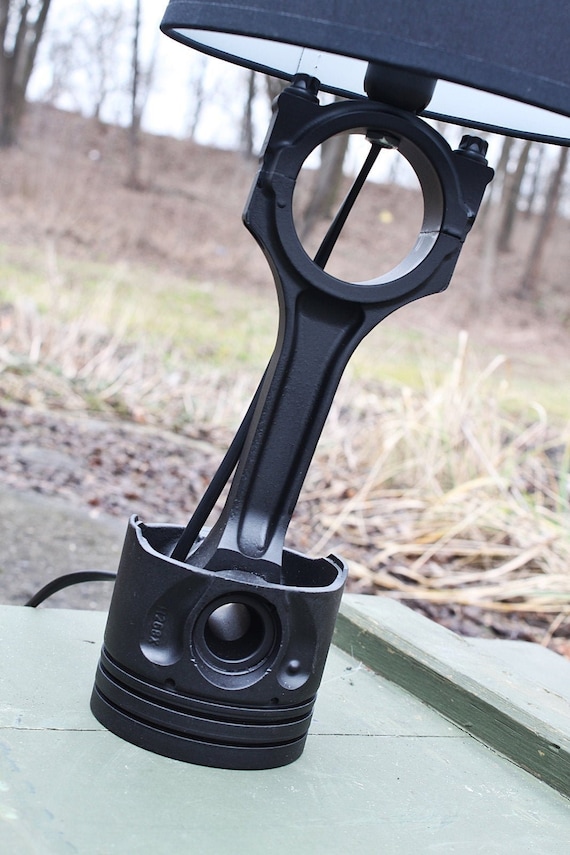This photograph captures a black lamp that appears to be slightly leaning to the right, placed outdoors on a green-painted wooden crate. The lamp has a mechanical, futuristic design, resembling a wrench with bolts and circular cut-outs. The base is black, resembling the bottom of a canister, with a matching black cord running down. The bottom part of the dark blue lamp shade is visible in the upper right corner. The setting is a natural outdoor environment with patches of green grass, brown dirt, and a backdrop of bare trees, suggesting an autumnal season. The background is slightly blurry, showing various plants and dead leaves, contributing to a rustic and somewhat mysterious atmosphere, illuminated by the soft light of a gray daytime sky.